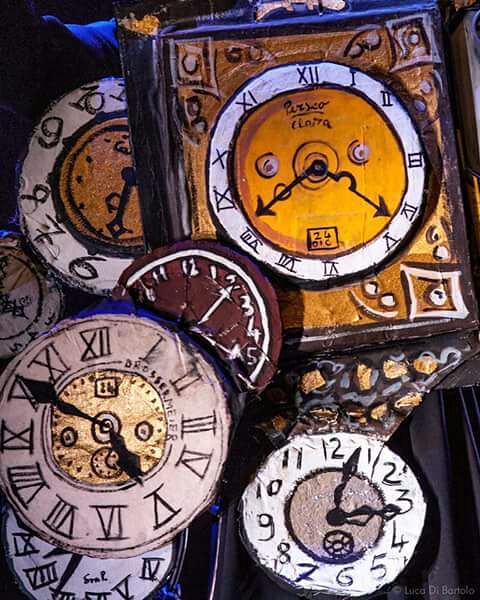This artwork is a detailed, surrealist painting of seven distinct clock faces featuring diverse designs, colors, and numeral styles. The largest and most prominent clock, situated at the top, has a golden yellow, square base with intricate geometric patterns, a round face with Roman numerals, and black hands with a distinctive hop in the hour hand. To its right, a square gold clock with a round face, Roman numerals, and black hands shows the time as 8:18.

Moving to the upper left, partially obscured by darkness and a hint of blue that might suggest an arm, another clock displays basic, childlike numerals, white along its outer edge, and a gold-orange center with dots marking the hours. This clock reads approximately 6:30. Just below this clock, a brown clock with white rudimentary numbers indicates 2:25.

In the center, slightly to the right, another clock features Roman numerals, a gold center, and black hands showing 4:50. Below it, a white clock with black hands and numbers, plus a small round dial beneath its main hands, indicates just after 3:00. On the far right bottom side, there's a white clock with Roman numerals and a gold center, indicating the time as 8:36.

The artwork's various shades of white, gold, black, and brown, combined with the mix of Roman numerals, basic childlike digits, and traditional English numbers, contribute to a vivid and eclectic timepiece tapestry, evoking a surreal and timeless ambiance.